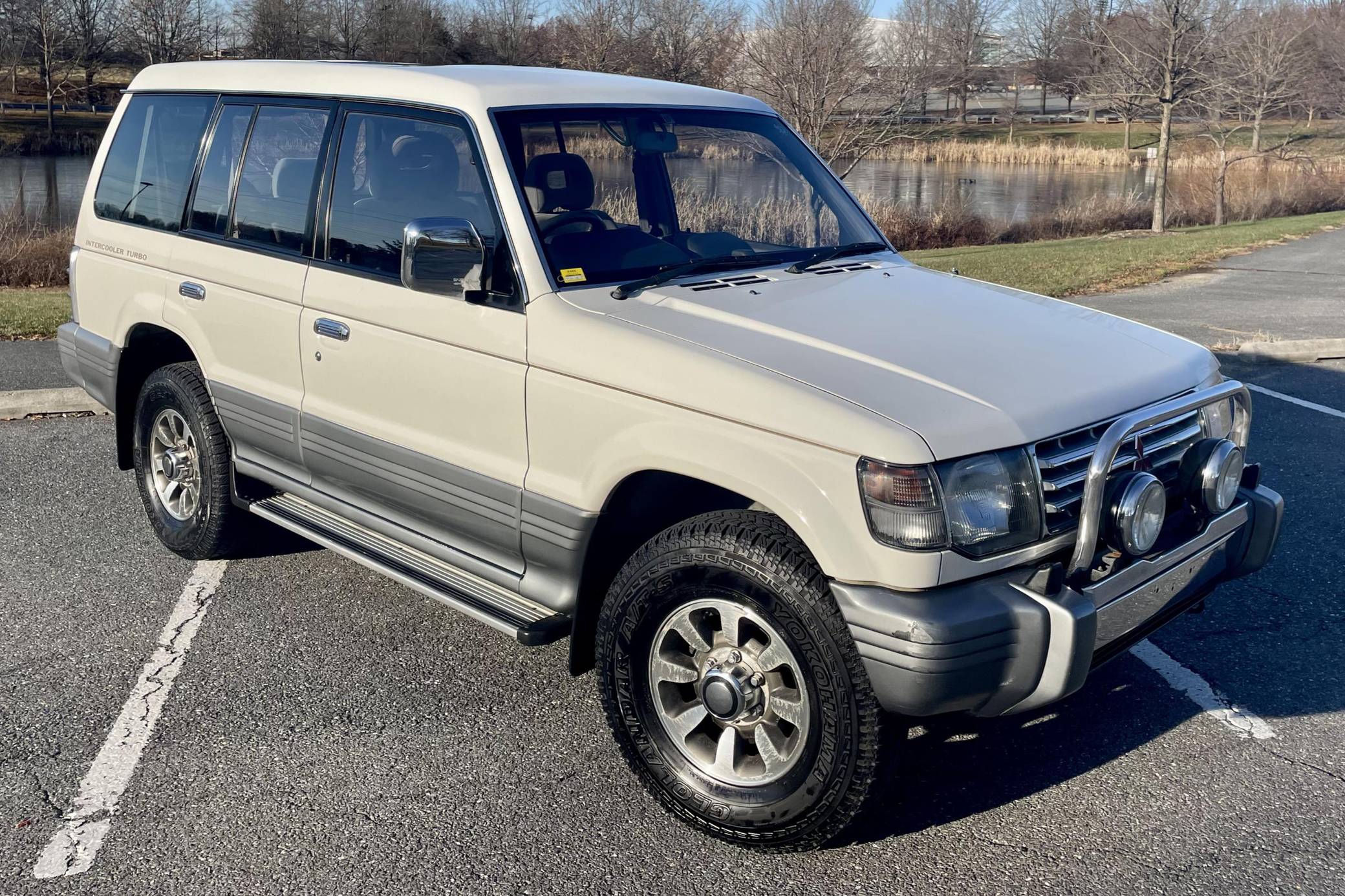The photograph features a white and silver SUV, possibly a Toyota RAV4, parked prominently in an outdoor parking lot. This mid-to-full sized, four-wheel drive vehicle is distinguished by its aluminum rims with heavy-duty tires and a rugged front grill bar outfitted with two large, circular floodlights, complimenting square-shaped headlights and standard turn indicators. The SUV's design includes a roof and upper side panels in white, transitioning to a silver hue two-thirds down the sides, along with a practical sideboard for entry. The vehicle appears spacious, with visible front and rear seats and windows extending to the back, one of which slides open.

The parking lot setting features the SUV angled across three parking spaces, its shadow cast to the right of the image. The background reveals a serene lake or pond lined with tan reeds and scattered trees bare of leaves, suggesting a winter scene. There is a mix of brown and green grass patches surrounding the area. A large building, mostly blocked by the trees, is also visible in the distance, adding depth to the outdoor landscape.